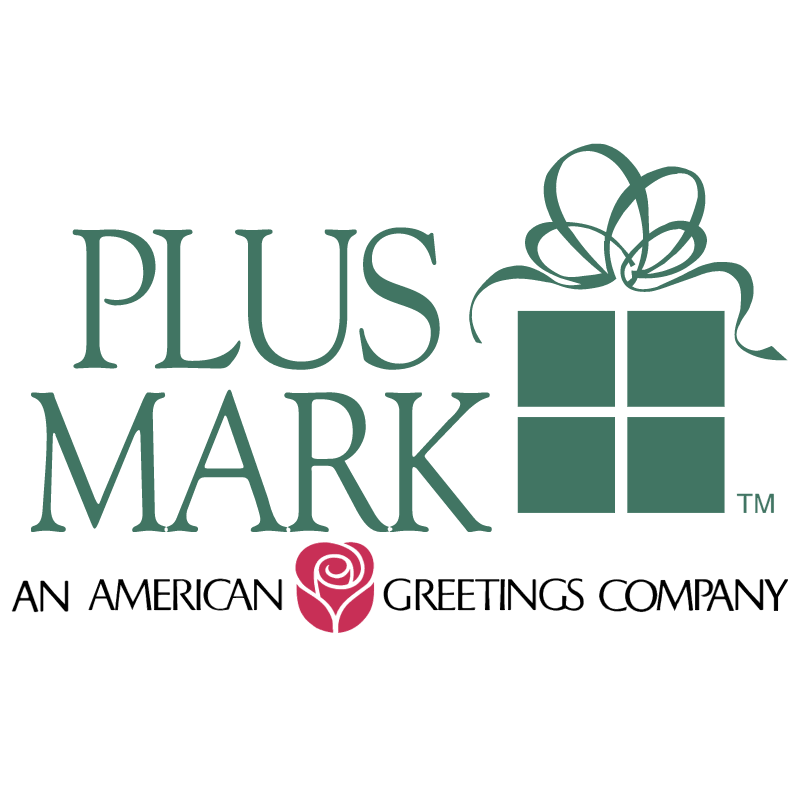This advertisement for an American greetings company, believed to be a card company, showcases a clean, modern design on a white background. Dominating the left side is the bold green text "Plusmark" in Arial font, with "plus" positioned above "mark." To the right, a gift box icon is prominently featured. This icon is creatively designed using four green blocks arranged to form a square, intersected by white lines to give the appearance of gift wrapping. Atop the box are wavy lines representing a ribbon. In the bottom right corner of the gift box, the letters "TM" indicate a trademark.

Running along the bottom of the image is the text "an American Greetings company" in black, uppercase letters. This text is interrupted by an icon of a red rose positioned between "American" and "Greetings." The overall composition, balancing modern simplicity with traditional elements, suggests an inviting and professional image aimed at attracting potential customers to explore the brand's offerings.